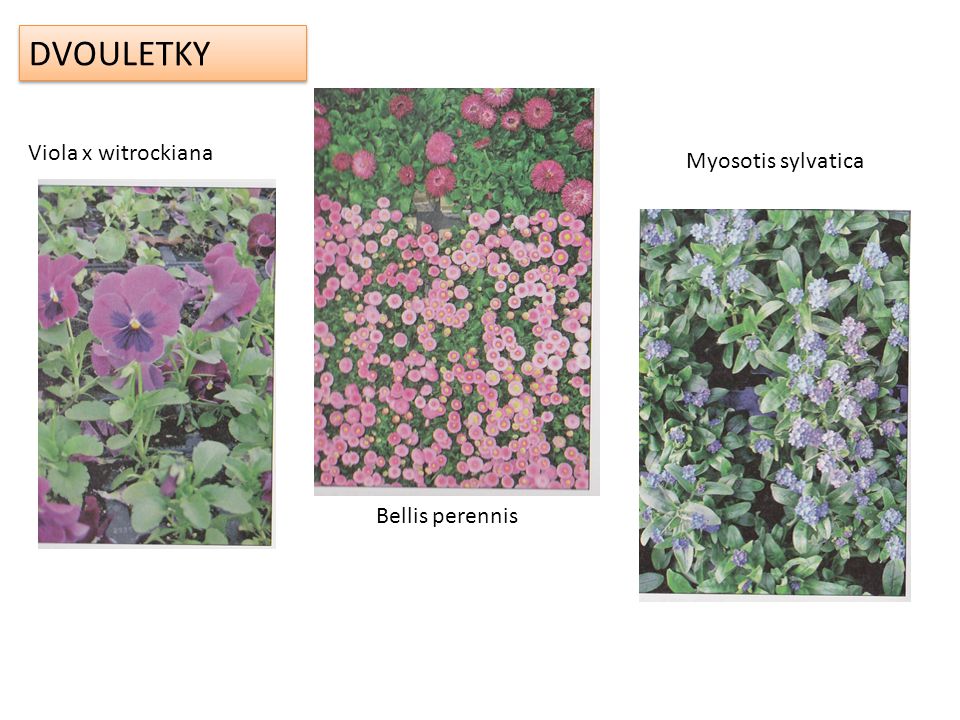This image showcases three distinct botanical illustrations, each labeled with their respective Latin names. On the far left, labeled "Viola X Wittrockiana," we see a plant featuring small green leaves and vibrant purple flowers, with darker purple centers. The middle image, labeled "Bellis perennis," depicts small, disk-shaped pink flowers with yellow centers resembling a ham and cheese sandwich, surrounded by some green foliage. Above, there are additional purple flowers. The image on the right, labeled "Myosotis sylvatica," presents green leaves and delicate purple flowers, resembling lilies. At the top of the image is a text box with the unclear inscription "D-V-O-U-T-L-E-T-K-Y." The collection showcases the diversity in flower types and plant families, with each plant featuring unique coloration and floral structures.